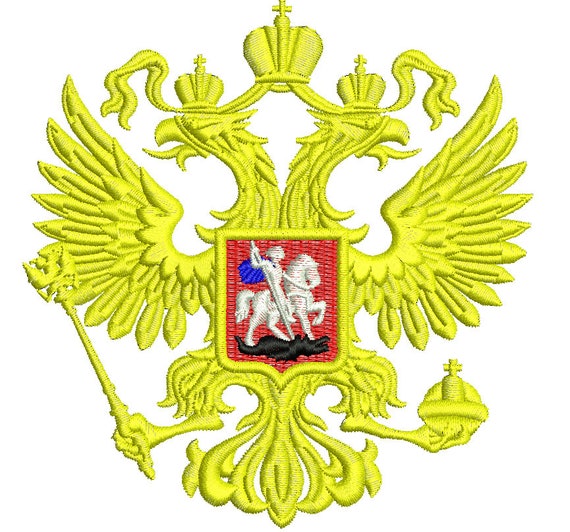The image features a large, yellow-colored medieval-style crest set against a plain white background. At its pinnacle, a crown adorned with a small cross sits majestically. Two additional crowns, each also topped with a cross, flank the central crown to the lower left and right. The crest's design incorporates wings on either side, with pointed tips extending outward, giving it an imperial feel. At the lower section, disembodied arms are depicted, with the left holding a spear and the right clutching a scepter-like container, also capped with a cross. Central to the larger crest is a smaller badge with a vivid red background outlined in yellow. This inset displays a white knight mounted on a galloping white horse, wielding a spear in his hand. The horse and rider are highlighted against small blue patches, enhancing the emblem's ornate and dignified composition.